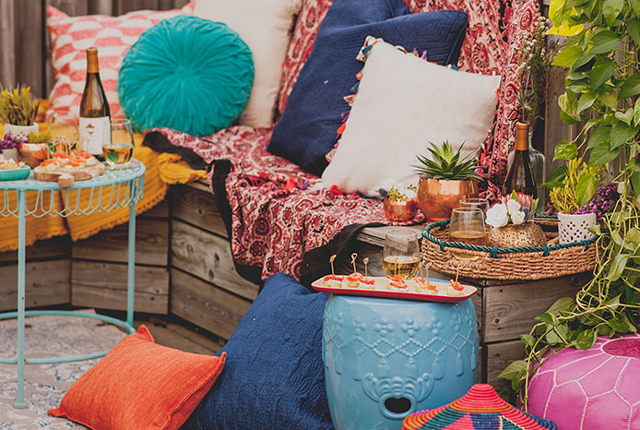The photograph captures a vibrant outdoor seating area, meticulously styled with a bohemian and eclectic aesthetic. A built-in wooden bench forms the central feature, covered with a red, white, and black paisley blanket and adorned with an array of pillows in diverse colors and patterns, including white, dark blue, turquoise, cream, pink, and orange. Situated against a fence, the bench is accompanied by a light blue metal table in front, holding wine, charcuterie, and a small plant. 

To the right, a wooden table supports a circular serving tray with more wine glasses, a bottle, and tiny potted plants. Walking into the scene, one encounters additional décor including a blue ceramic vase with appetizers. The colorful setting is further decorated with lush green vines and potted plants, injecting life into the vibrant assemblage of textiles and pottery. The image, likely meant for a home design advertisement, reflects a cozy, inviting space perfect for a gathering, emphasizing comfort and color harmony in an outdoor patio environment.